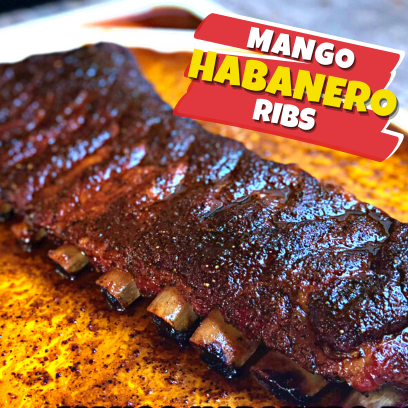The advertisement features a close-up image of a rack of about 10 Mango Habanero Ribs, prominently displayed on a yellow, round plate. The ribs appear to be thoroughly barbecued, showcasing a rich, brownish-red glaze that indicates they are well-seasoned and marinated. Visible spices and the distinctive mango habanero sauce add a vibrant touch to the dish. The image itself is zoomed in to emphasize the succulent details of the ribs, with the bones sticking out slightly on one side. In the upper left-hand corner, the text "Mango Habanero Ribs" is presented, with "Mango" and "Ribs" written in white, and "Habanero" highlighted in yellow, enhancing the spicy and exotic appeal of the dish.